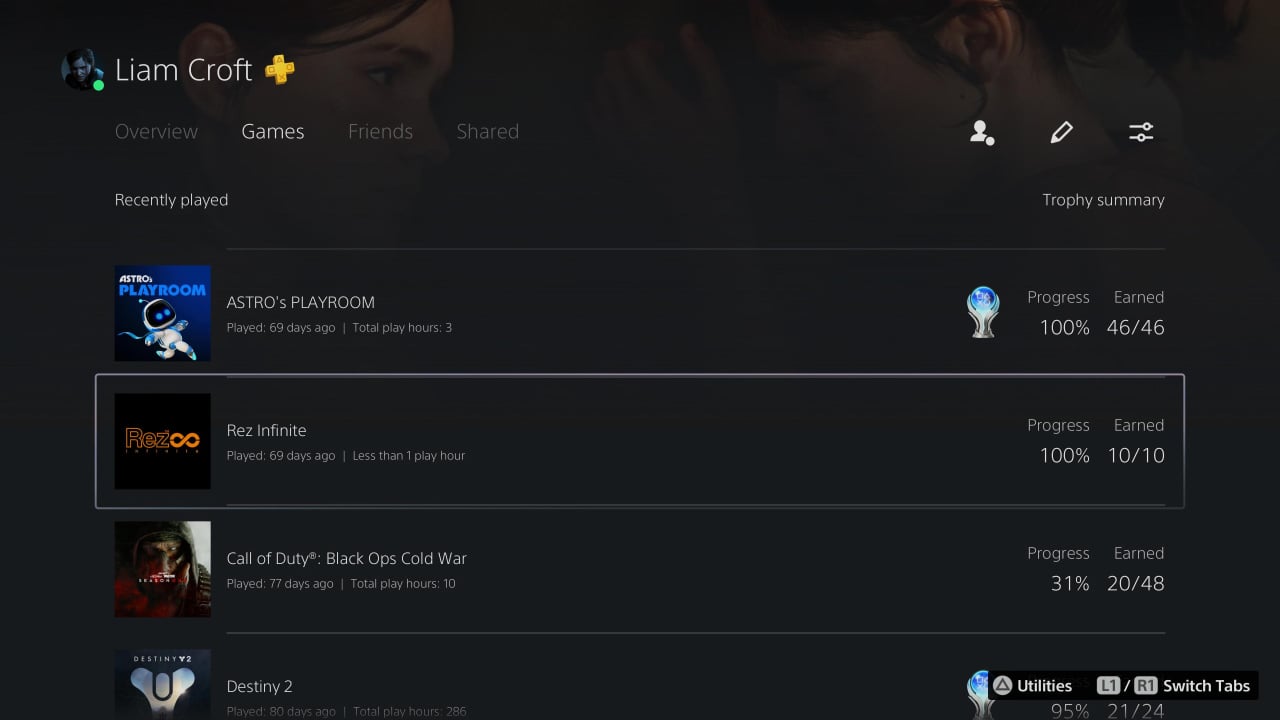Screenshot of a gaming website featuring a realistic animated background with two dimly lit, AI-generated girls looking at each other. In the top left corner, the username "Liam Croft" is displayed, accompanied by a golden plus sign. Below the username, navigation options are visible, with "Overview" and "Games" listed side by side. The "Games" option is highlighted, suggesting it is currently selected. Underneath these options, a section titled "Recently Played" is showcased. Within this section, an entry for "Astro's Playroom" is displayed, complete with an image of a little man in a spacesuit. To the right of this image, the game's progress is indicated as 100%.